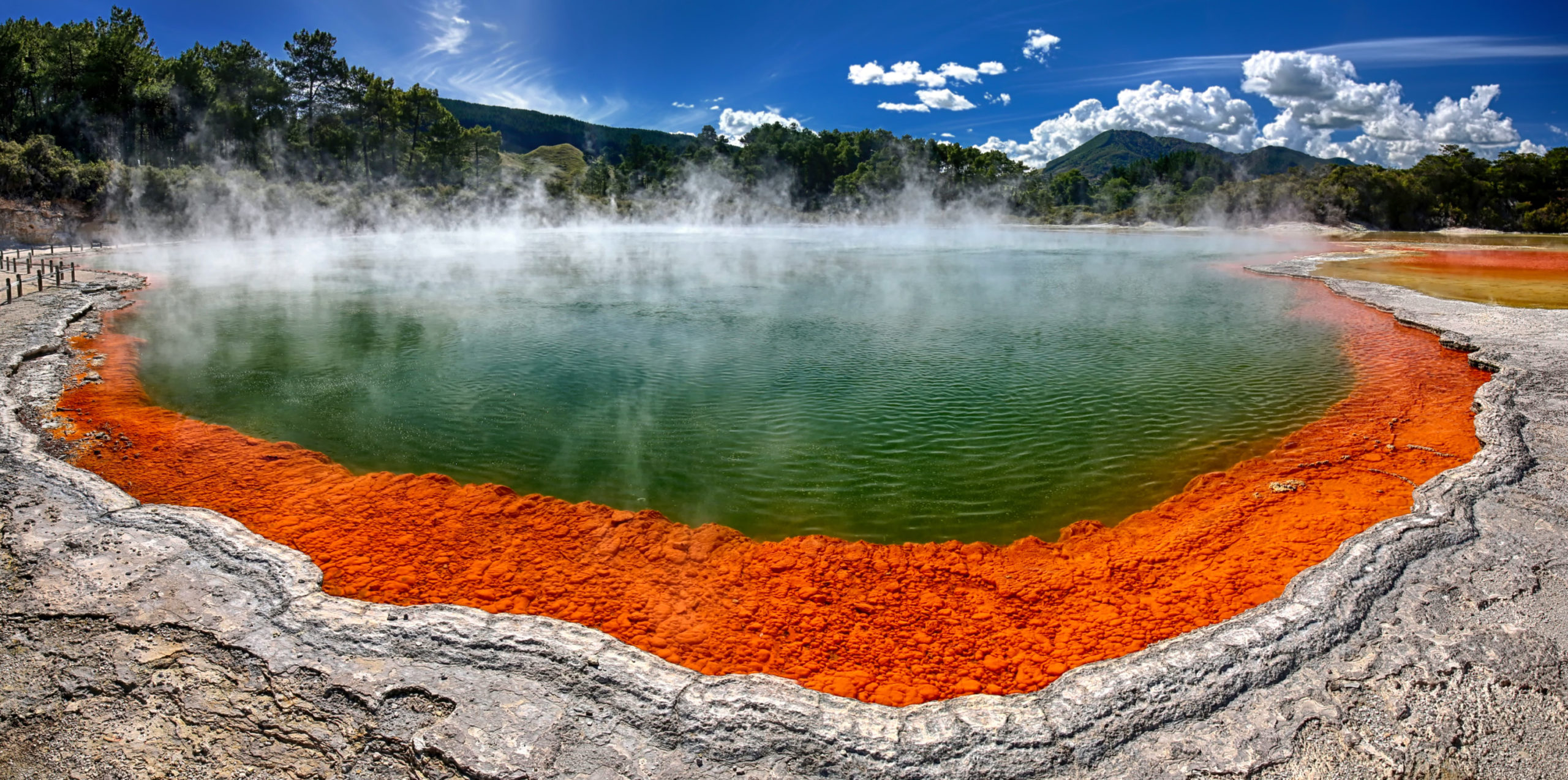The image captures a close-up of a vast, steaming hot spring with water that shifts from a murky green near the foreground to a foggy blue towards the center. Gray, ridged rocks surround the pool, which is emitting steam, suggesting high temperatures. Just before the rocky shoreline, there is a dense layer of orange-red soil floating on the water's surface. The hot spring stretches up to the horizon where slightly raised, rolling hills begin. These hills are covered in a lush, dark green forest with trees concentrated more to the left side. Above the hills, a partially cloudy sky takes over, with clouds more abundant on the right side and sunlight filtering from the left. The serene background hints at an untouched natural landscape, accentuating the scenic beauty and the heat of the foreground pool.